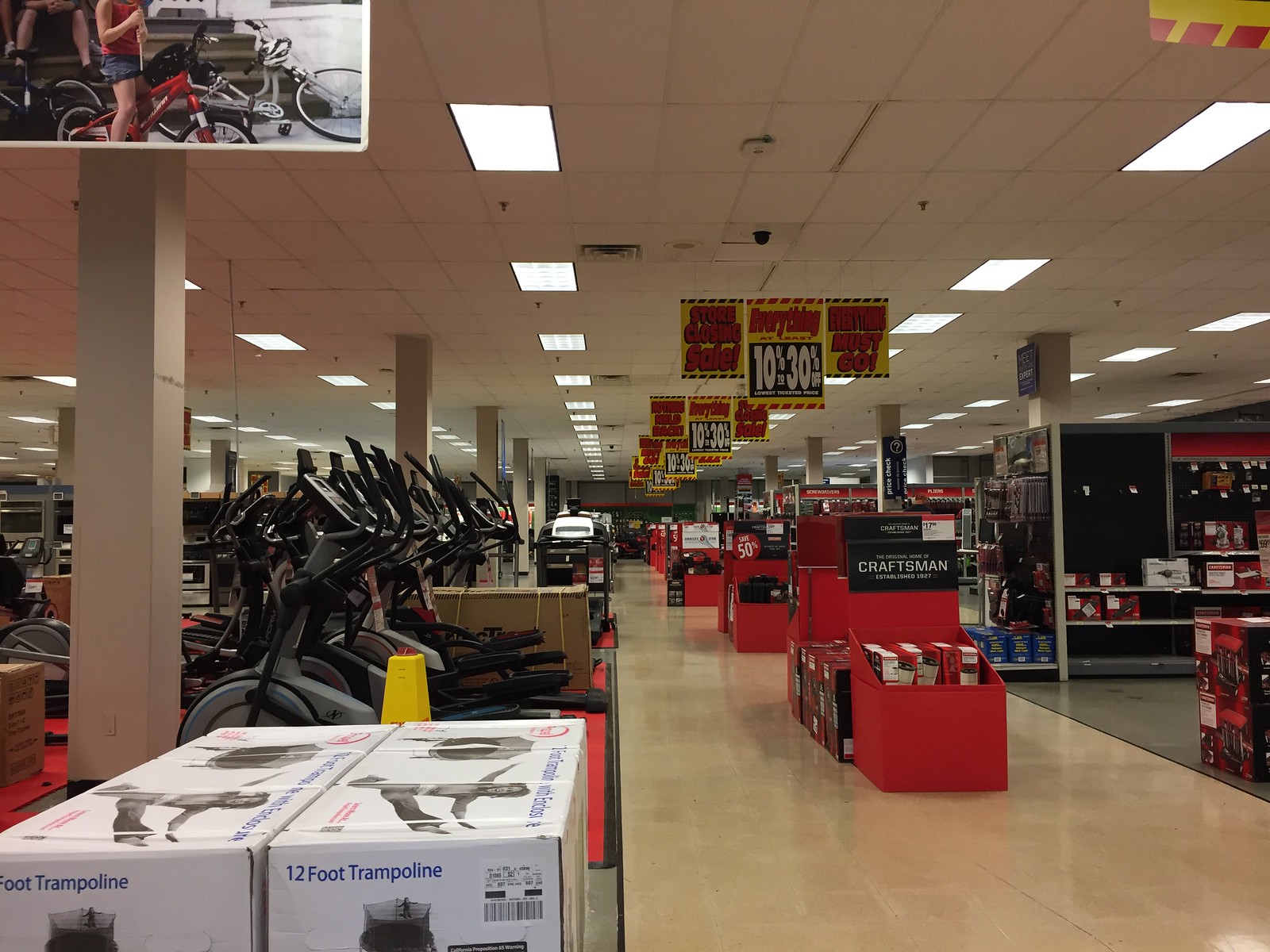The image depicts the interior of a large retail warehouse store, resembling a Kmart, Walmart, or Target. The wide aisle features multiple displays and items for sale. 

To the left, there are several exercise bikes prominently displayed on a red-carpeted black platform. In the foreground, large white boxes labeled "12-Foot Trampoline" in blue text dominate the scene. Each box features an image of someone jumping on a trampoline.

Towards the back of the aisle, various other items are visible, though difficult to distinguish clearly. It seems there might be a riding lawnmower in the distance. The middle section of the aisle is lined with red shelving units, with the first shelf showcasing "Craftsman" products, indicated by white text on a black background.

The yellow sale banners hanging from the ceiling announce discounts, with one reading "10 to 30% off" in white text on a red background within a blue box. Another sign suggests urgency with phrases like "Hurry" and "must go."

The ceiling is white, with built-in lights illuminating the store. On the right side, more shelves are stocked with various items. The floor is a glossy beige linoleum transitioning to gray tile as the aisle progresses.

An insert at the top of the image features a white bike and a red bike, with a person in blue shorts and a red top sitting on the latter. In the background, a customer appears to be examining the bikes. The overall scene is busy, well-lit, and filled with a variety of goods characteristic of a large retail store.